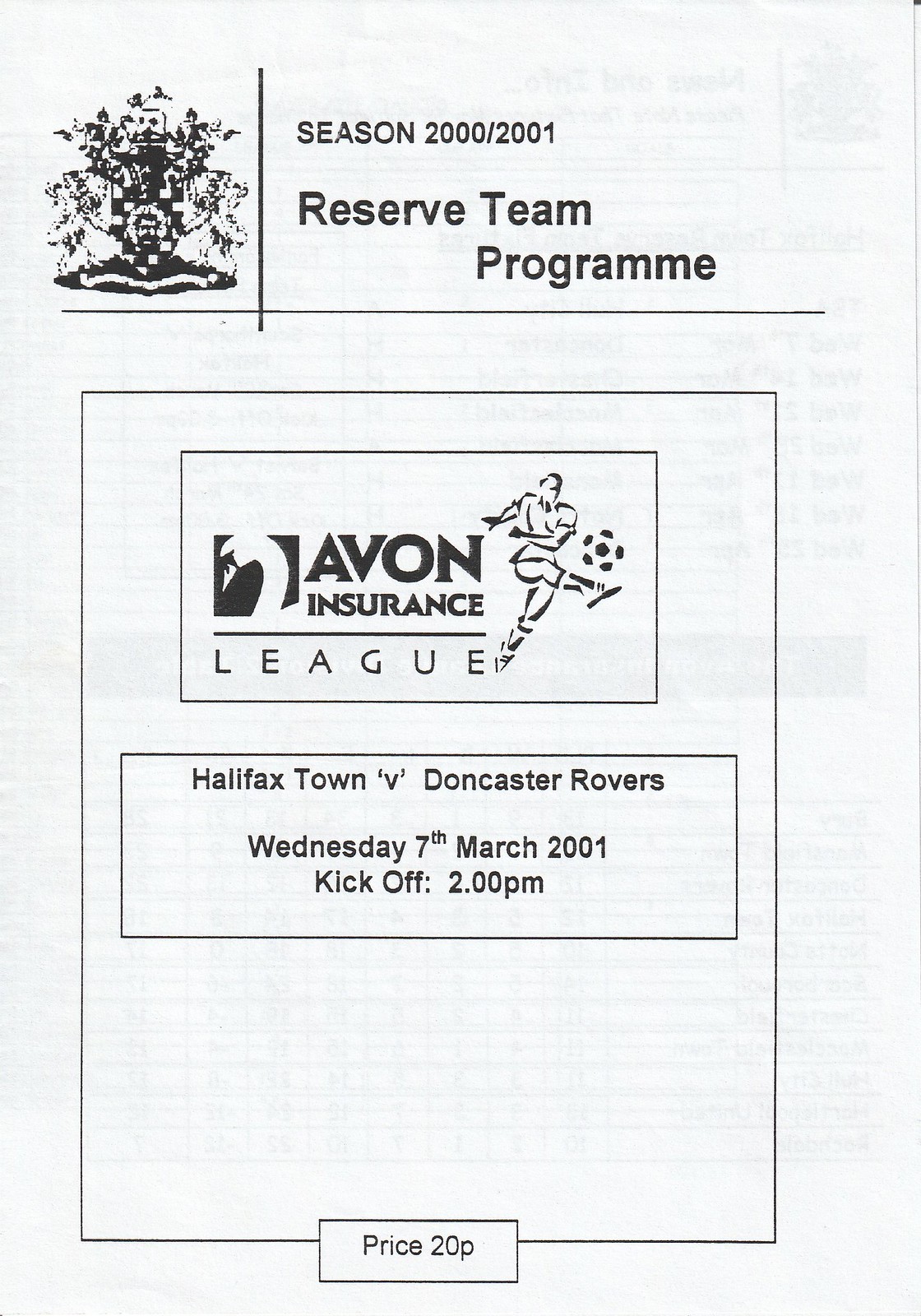This is a detailed description of the front page of a soccer club's program for the 2000-2001 season. The top of the page reads "Season 2000-2001" on the right, accompanied by a logo on the left that depicts a tree and the image of a man. Directly below this, the text "Reserve Team Program" is prominently displayed. The design includes a rectangular box containing an advertisement for the "Avon Insurance League," featuring a logo with a white swoosh on the left and a soccer player kicking a ball on the right. Below this advertisement, another box provides the match details: "Halifax Town vs. Doncaster Rovers, Wednesday 7th of March 2001, kickoff 2 p.m." At the very bottom of the page, a small box indicates the price of the program as "20 pence." The page has a simple black and white color scheme, with brown lettering.